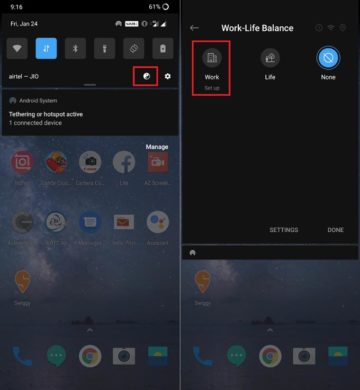The top left of the image features a square with a black background containing several square icons. The first icon to the left is a Wi-Fi symbol with a medium gray background and light gray icon. Next to it, there is an icon with a downwards and upwards arrow on a blue background, indicating it is selected. To the right of this, there's a light gray Bluetooth icon followed by a flashlight icon. There are two more icons next in line, but they are indiscernible.

Below this area, in the center, there is another icon that is white and highlighted within a red square border, though the specific details of the icon are unclear. The image also shows a traditional Android notification beneath these icons.

The wallpaper of the screen appears to depict either water or the sky, enhancing the visual aesthetics. Among the app icons on the wallpaper, there's the InShot app icon, next to which is the Candy Crush icon, followed by an app that resembles a camera. To the right of these, the Facebook app icon is visible along with an app that has an orange video camera icon. 

Towards the bottom of the screen, a dock holds several icons starting with a blue phone icon, a green messaging icon that could be WhatsApp, the Google Chrome icon, and a camera icon. Additionally, there’s an icon that may suggest an image with a dark blue bottom and a light blue top, potentially representing a sky with a sun.

At the top of the image, the text "Work-Life Balance" is displayed in white. Below this, a red rectangular area is highlighted with the word "Work" and an accompanying building icon, alluding to a work-related context in the interface.